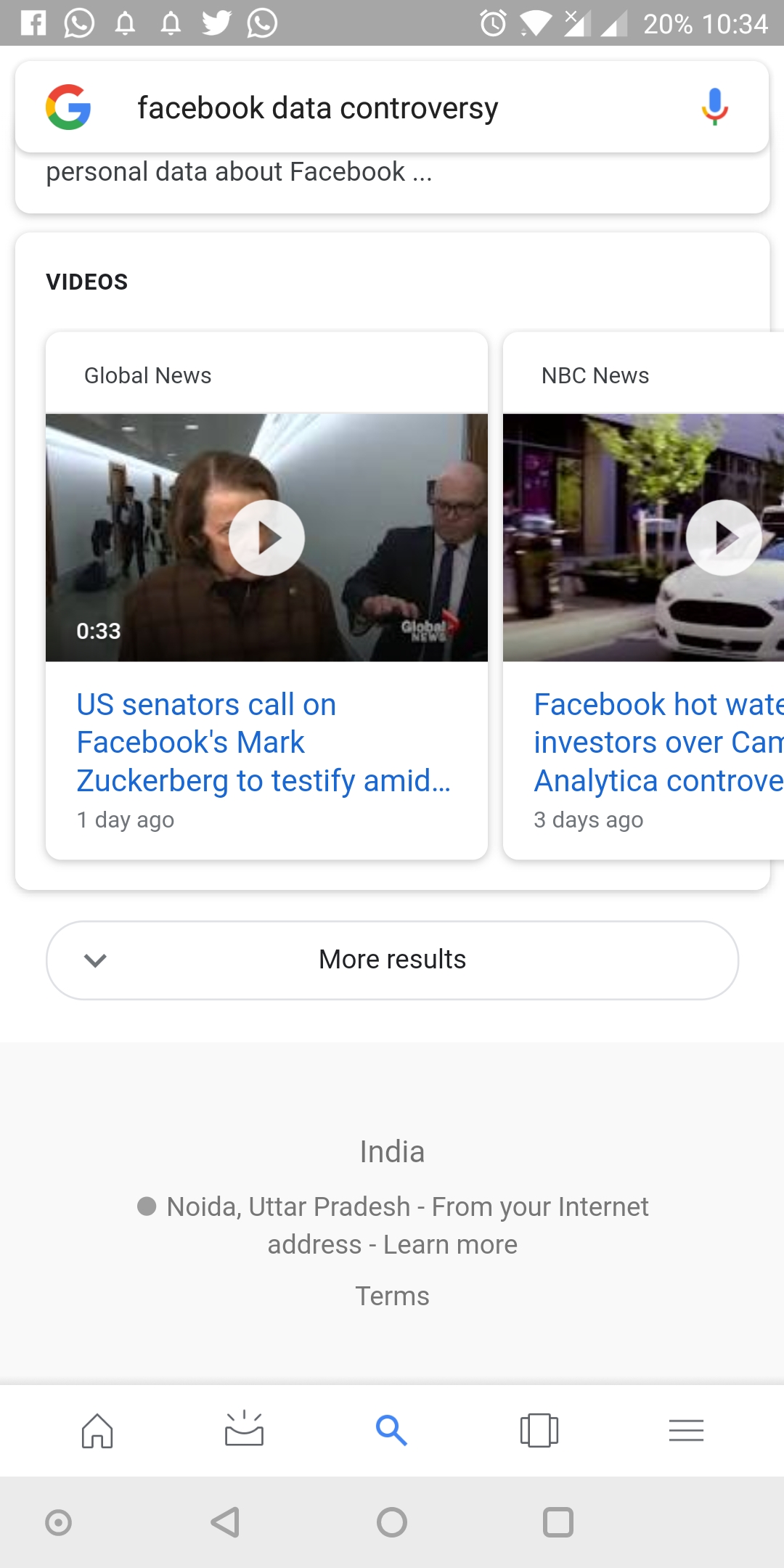The screenshot shows a cell phone interface with a white background and grey text. The screen captures various app icons including Facebook, WhatsApp, Snapchat, and Twitter. The phone displays the current time as 10:34 and has a battery level of 20%. There are indicators for phone signal issues, WiFi, and airplane mode.

At the top, there is a Google search bar with the "G" logo, where a user has searched for information related to the "Facebook data controversy." The search results include two video thumbnails: one discussing US Senators questioning Mark Zuckerberg, and another from NBC about Facebook facing criticism. Additional results are displayed below these videos.

In grey text, it mentions "India" and "NOLA ATAR PARASH" along with an option to learn more about terms related to the user's internet address. At the bottom of the screen, there are various icons: a house, a crown with spikes, a magnifying glass, a book, and three horizontal lines. To the left, a button with a circle and a dot in the middle is visible, along with a left-pointing arrow and another circle.

The user's commentary also mentions some personal data related to Facebook and wishes everyone a good day, ending with "world star."